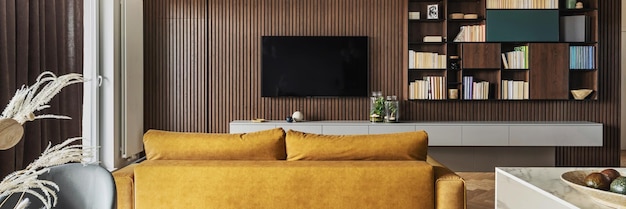The image depicts a modern living room or lounge area, probably in an apartment or condo. The walls are adorned with sleek, textured paneling of thin vertical lines, giving a sense of depth and contemporary style. A flat-screen TV is wall-mounted, slightly off-center, with a white shelf underneath holding two decorative jars. To the right of the television, a large built-in bookshelf houses an eclectic mix of books, most with their pages facing outward, complemented by several small vases and a picture. 

In the foreground, a mustard yellow sofa is seen from behind, its two large cushions peeking above the backrest, serving as the primary seating for television viewing. A marble-topped table with a decorative bowl containing round ornaments is visible, adding a touch of elegance. To the left side, an artificial plant and part of a gray chair can be seen, along with brown curtains that likely frame a sliding glass door. The overall atmosphere is cozy yet stylish, blending modernist elements with personalized touches.